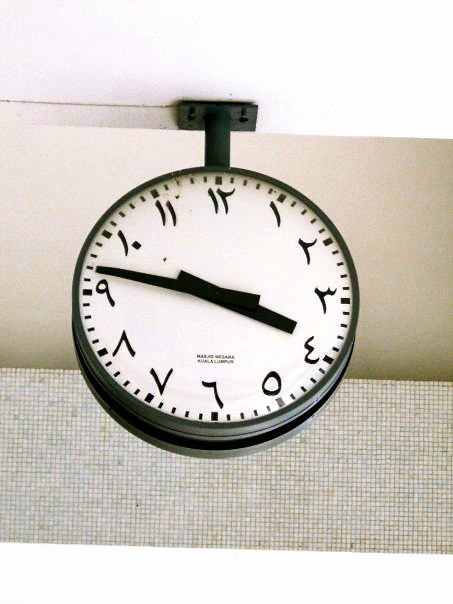This color photograph captures an analog clock mounted in a public indoor space, likely a train station given its double-sided design, suspended from the ceiling with a metal frame and bolted in with two screws. The clock, which has a bold black rim, features a stark white face with black minute and hour hands. Its numerals appear to be in a foreign script, possibly Arabic or Hebrew, making them largely unreadable to those unfamiliar with these scripts. Despite this, the clock adheres to the typical layout with 12 distinct symbols marking the hours. The setting has a gray, slightly textured background, contributing to an older, non-modern aesthetic. The hands on the clock show the time to be about nine minutes to four.